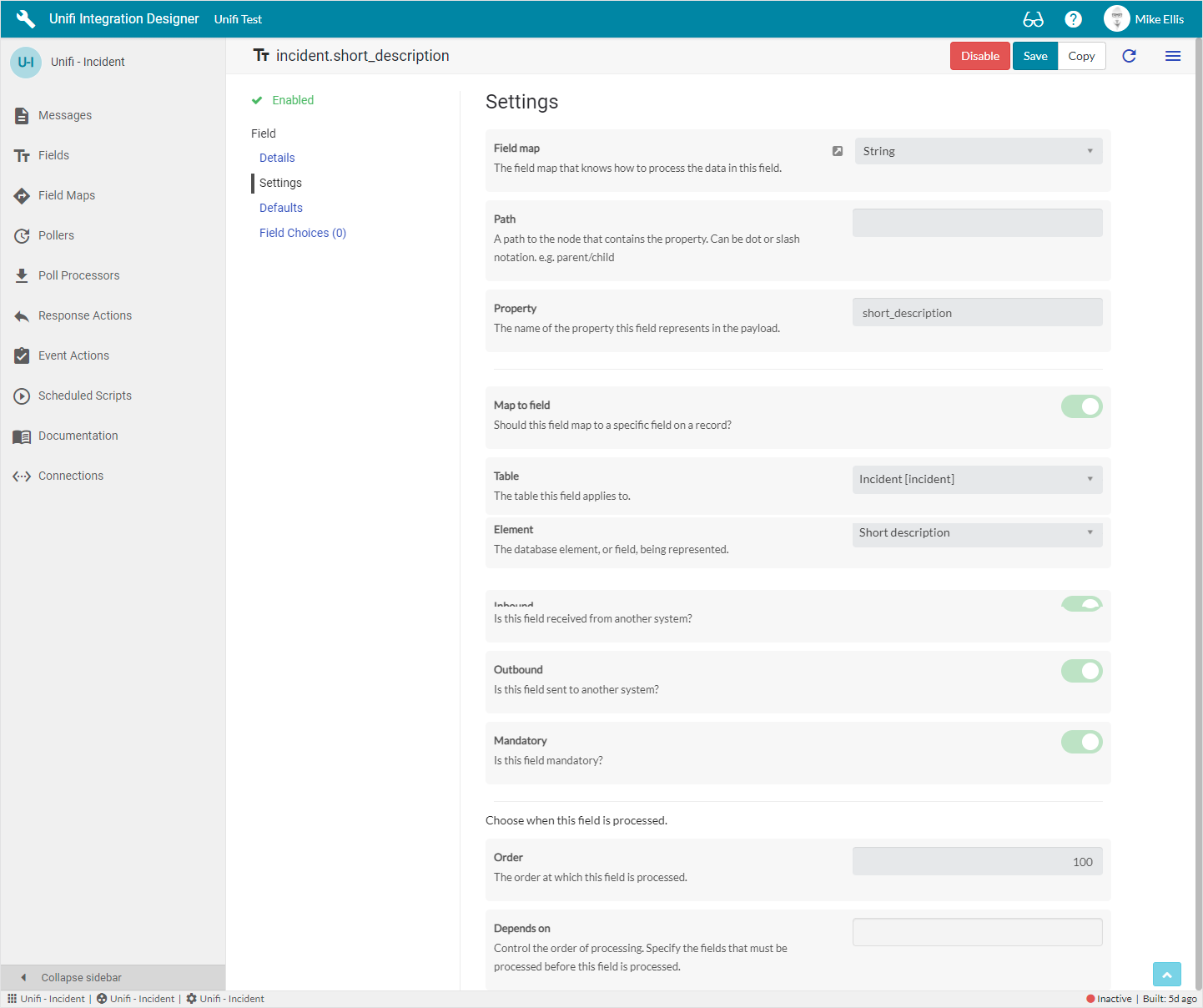This image captures the settings page of a website or application, presented in a roughly square format. A prominent gray vertical line runs down the right side, framing the image. The page header is highlighted with a greenish-teal rectangular border stretching across the top, featuring white text. On the left side of this header, a wrench icon precedes the text "Unify Integration Designer," followed by a blurred word "Test." Further right, there are icons of sunglasses and a white question mark with green font inside. A white circle displays the name "Mike Ellis."

Below the header, a green circle with dark green text reads "UH Unify Incident." Above the main section, there are three buttons: an orange "Disable" button, a green "Save" button, and a white "Copy" button.

The primary content area features a white background with black text, headed by the title "Settings." This section includes various gray boxes designed for modifying settings. On the left side, a vertical border contains options, each with gray text and icons. These options include Messages, Fields, Fields Maps, Pollers, Poll Processors, Response Actions, Event Actions, Scheduled Scripts, Documentation, and Connections, among others. This detailed layout provides a comprehensive view of the settings interface, highlighting the functionality and navigational elements available to the user.